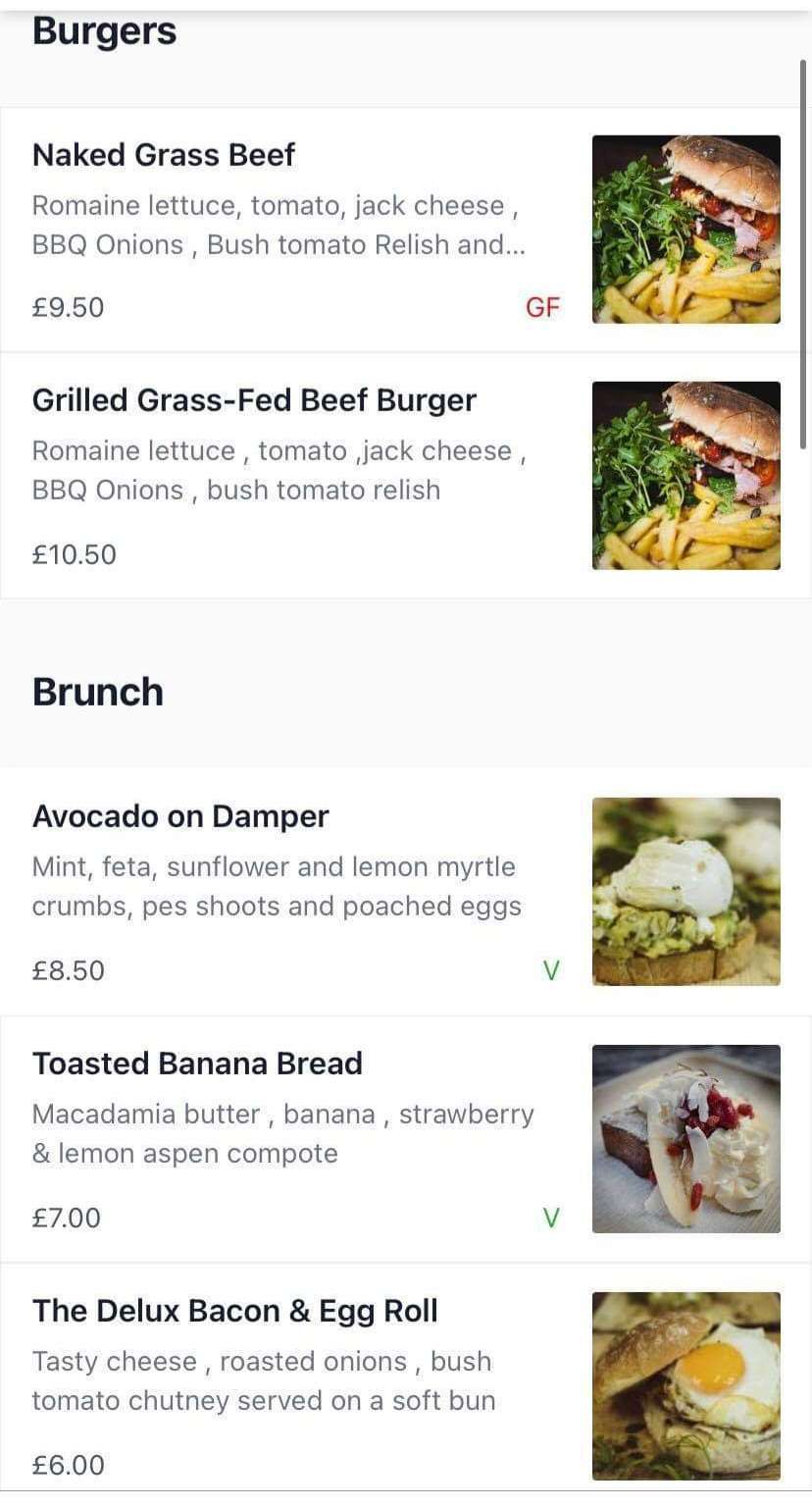The online menu from the virtual restaurant is displayed against a white background, with all text in black for clear readability. At the top left corner, the category "Burgers" is prominently featured.

1. **Naked Grass Beef Burger** - Priced at £9.50 and categorized as GF (Gluten-Free), this burger includes romaine lettuce, tomato, jack cheese, BBQ onions, and poached tomato relish. The accompanying image shows the burger served with crispy yellow fried chips and a side of fresh green lettuce.

2. **Grilled Grass Beef Burger** - This burger costs £10.50 and shares the same ingredients as the Naked Grass Beef Burger: romaine lettuce, tomato, jack cheese, BBQ onions, and poached tomato relish. It is also served with fries, as shown in the image.

Further down, the menu introduces the "Brunch" section:

1. **Avocado on Damper** - For £8.50, this dish comes with mint, feta, sunflower seeds, lemon myrtle, crumbs, peaches, and poached eggs. Its image is shown on the right and is marked with a green "V" indicating it is available on weekends.

2. **Toasted Banana Bread** - Priced at £7.00 and classified as vegan, this item features macadamia butter, banana, strawberry, and lemon aspen compote.

3. **Deluxe Bacon and Egg Roll** - This final brunch item costs £6.00 and is made with tasty cheese, roasted onions, poached tomato chutney, and is served on a soft bun. The corresponding image depicts a roll with yellow and white egg.